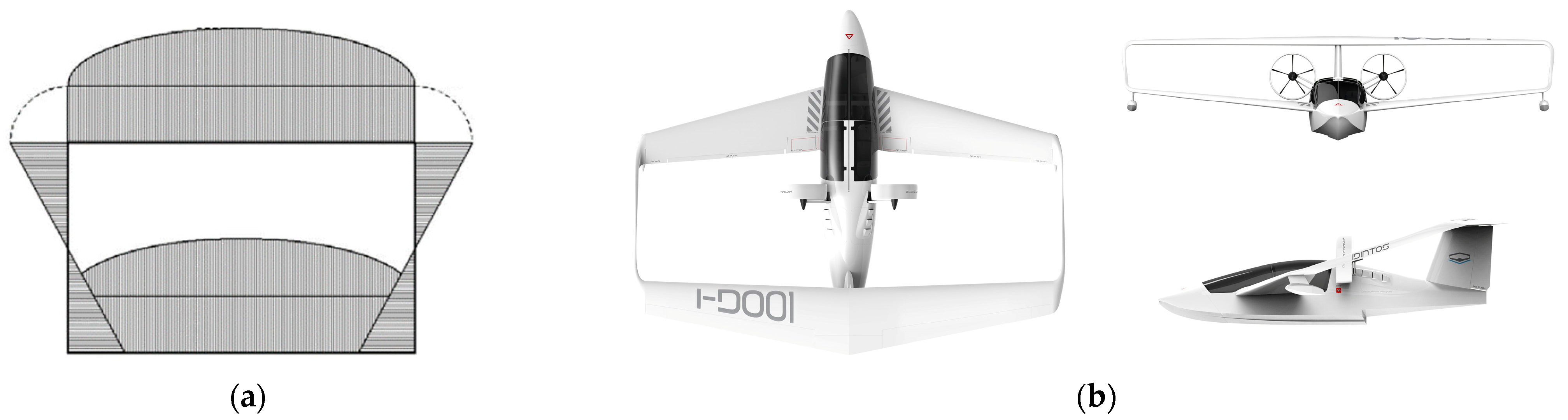The image is a composite showcasing multiple perspectives and details of a sleek, futuristic small airplane. The primary section, labeled as Figure B, comprises three photographs depicting the all-white airplane: a top view, a front view displaying its two propellers, and a side view highlighting its sophisticated design. The aircraft features a see-through black glass cockpit, enhancing its modern appearance. In the secondary figure, labeled as Figure A, there is a line drawing or schematic of the airplane with intersecting lines, possibly illustrating a complex aspect or a different model. The drawing reveals a unique two-level wing system with the wings extending along the plane's length, and the body resembles a boat hull, suggesting it could be a sea plane. Notably, there is no visible landing gear, reinforcing this theory. The overall composition provides a comprehensive insight into both the aesthetic and possibly functional aspects of the airplane.